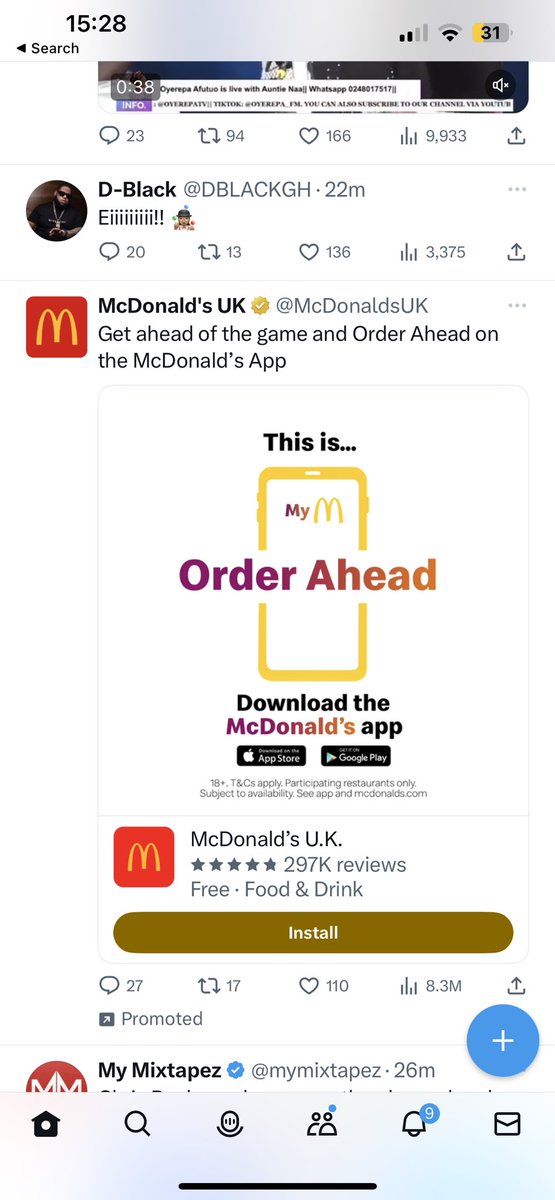This detailed caption captures everything mentioned with clarity and conciseness:

---

A screenshot of a smartphone displaying a Twitter feed. The top of the screen shows it is 3:28 PM (15:28), and indicates strong Wi-Fi and cell service with a battery level at 31%. The feed contains various tweets from individuals and organizations. At the very top, a partially visible, muted 38-second video is displayed. The first full tweet below the video is from a user with the handle @dblack, exclaiming "EI!!!!!!!!!". Following that is a promotional tweet from McDonald's UK, encouraging users to "get ahead of the game and order ahead on the McDonald's app," and includes an option to install the app. This advertisement is marked as promoted. Below this, there is a tweet from @MyMixTapes, an account verified with a blue checkmark, though the content of the tweet is cut off and unreadable.

---

This enhanced caption delivers a clear and descriptive overview of the screenshot, incorporating all the given details.